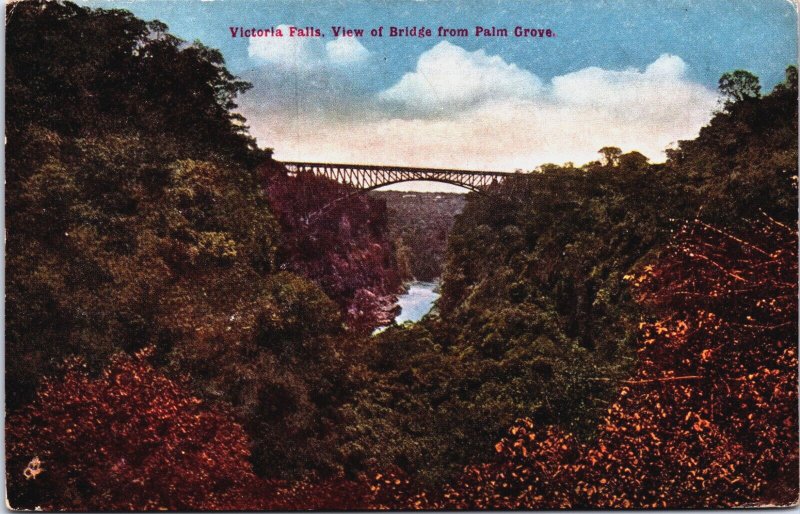The image is a vintage postcard titled "Victoria Falls, View of Bridge from Palm Grove." The postcard, which resembles those from the 1950s and has slightly curled and roughened corners, features a picturesque and colorized scene. Dominating the center of the image is a small suspension bridge with crisscrossing and vertical metal rods, and arched scaffolding underneath it, set against a beautiful blue sky dotted with fluffy white and pink-tinged clouds. The bridge spans above a stream that winds into the background, eventually merging into a tree-lined landscape. The foreground showcases trees with dark red to orange leaves, transitioning to various shades of green towards the back, from dark to yellowish-green. The image has a muted, somewhat blurred quality, enhancing its vintage charm. Although the town may be named Victoria Falls, no actual waterfall is depicted in the scene. Instead, the focus remains on the scenic bridge and surrounding natural beauty.